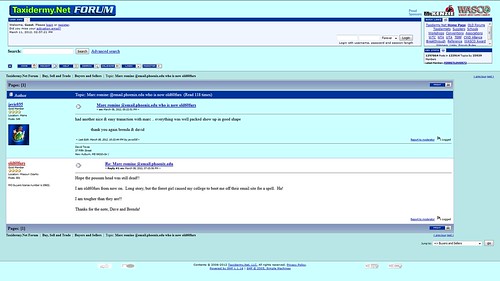This is a screen capture of the Taxidermy.net forum webpage. The background of the site is primarily blue, with a grey navigation box at the top, followed by a white content area, and another blue section at the bottom. The content displayed includes multiple discussion threads where people are conversing about various aspects of taxidermy. In one of the posts, a low-quality image resembling a crown is shown, accompanied by text that is difficult to read due to the image quality. Snippets of text below the image suggest topics like "mass something" and mention an additional piece that was easy to manage. Another post references something dried, indicating different users contributing to the discussion.

Along the right side of the webpage, there are two separate logos and various other elements. The left side features menus and quick links for navigating the site, including options like Forum, Schools, Resources, and various other informational sections pertinent to taxidermy enthusiasts. This comprehensive website, Taxidermy.net, serves as a hub for individuals interested in taxidermy to connect, share information, and discuss their craft.